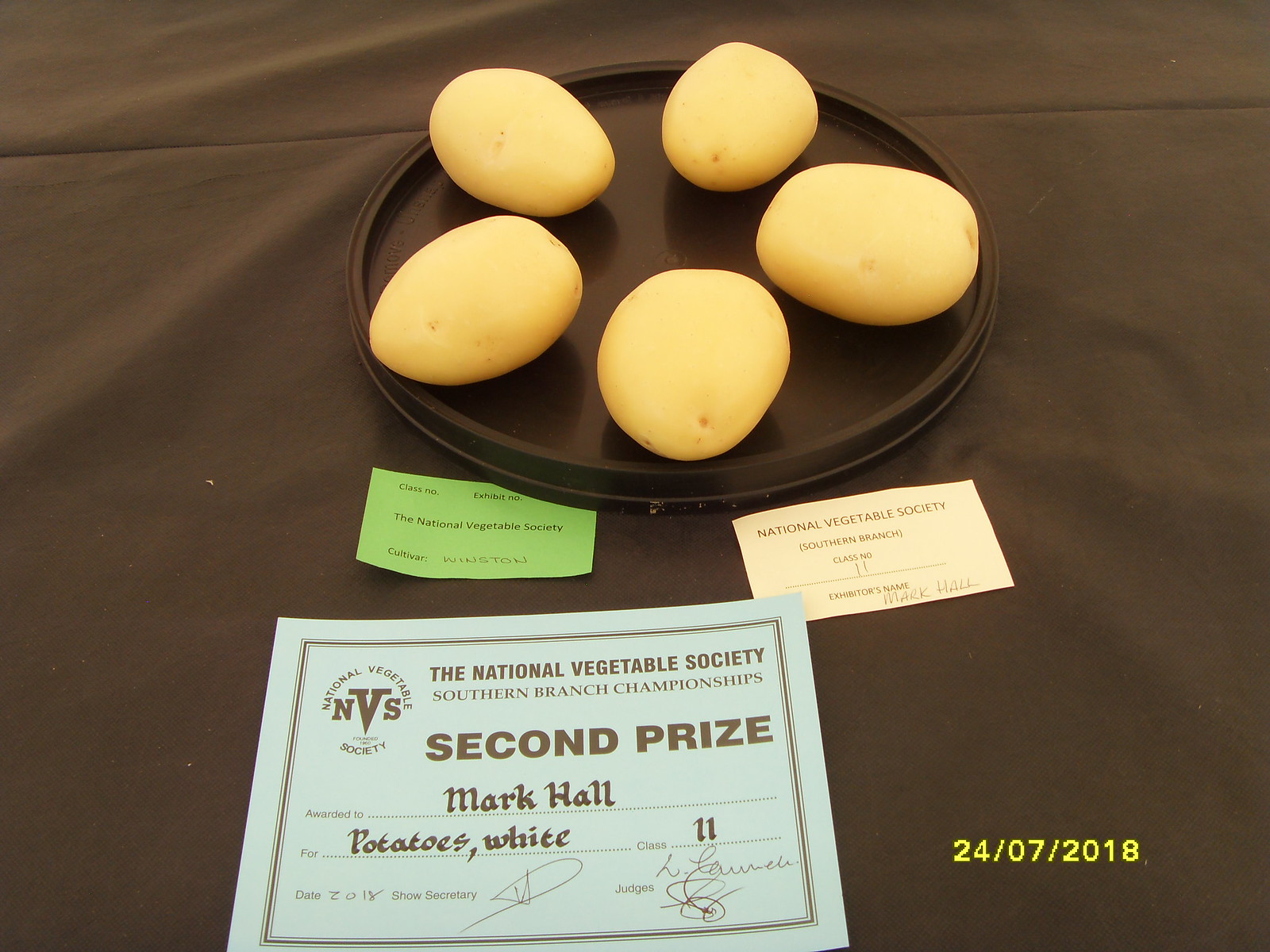In the image, five impeccably clean white potatoes are meticulously arranged on a flat platter, which sits atop a black tablecloth, clearly prepared for a contest display. These potatoes have earned accolades, evidence of which is prominently displayed through several cards placed on the table. The first card, green in color, is the exhibit number card affiliated with the National Vegetable Society. Next to it on the right, a white card from the National Vegetable Society Southern Branch denotes the competition class (Class Number 11) and the exhibitor's name, Mark Hall. Beneath these, a larger blue card proudly announces that Mark Hall secured second prize at the National Vegetable Society Southern Branch Championships for his white potatoes, Class 11. The details of this accolade include the date, July 24, 2018, which is also stamped on the photo itself, enriching the historical context of this event.